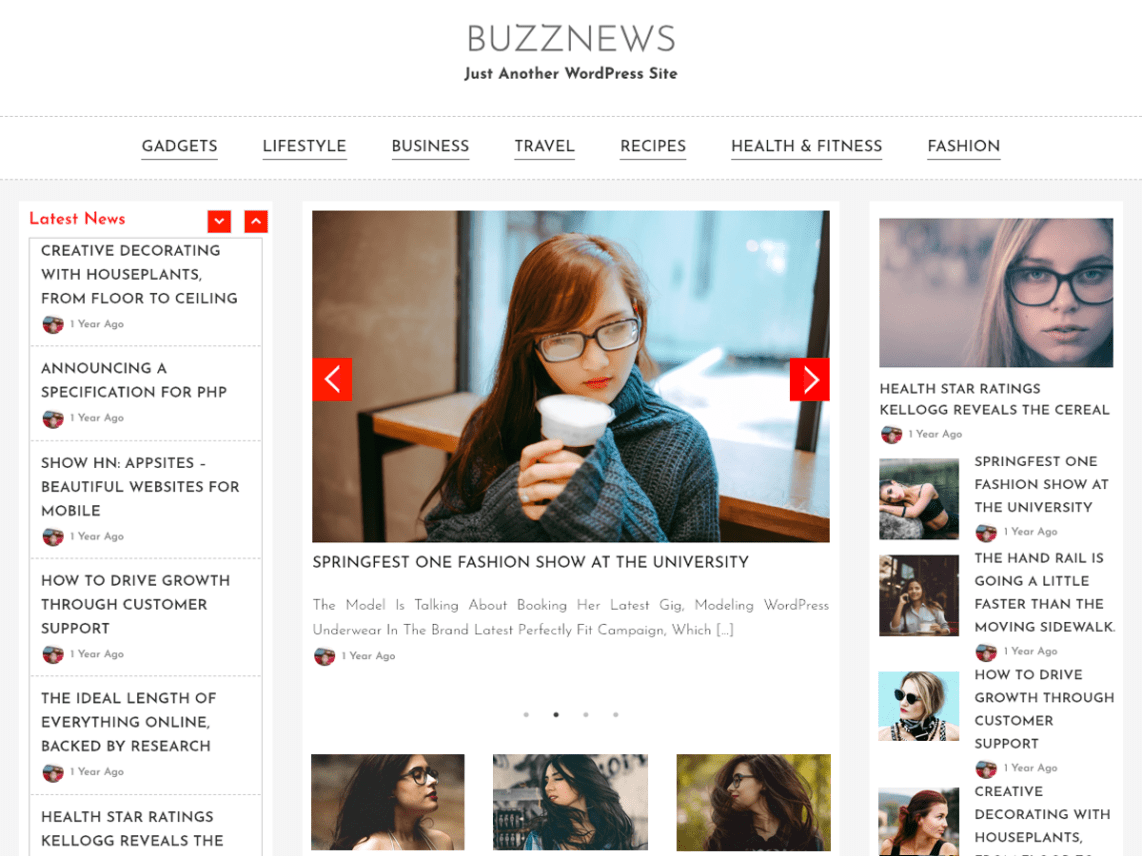The image depicts the homepage of a website titled "Buzz News: Just Another WordPress Site." The header of the site features a navigation menu with options such as Gadgets, Lifestyle, Business, Travel, Recipe, Health & Fitness, and Fashion. 

On the left-hand side, a sidebar labeled "Latest News" allows users to scroll through various articles. Some of the featured articles include: "Creative Decorating with Houseplants from Floor to Ceiling," "Announcing a Specification for PHP," "Show HN App Sites: Beautiful Websites for Mobile," "How to Drive Growth Through Customer Support," "The Ideal Length of Everything Online, Backed by Research," and "Health Star Ratings: Kellogg Reveals."

The central portion of the webpage is dominated by a main image that showcases a woman sipping what appears to be a latte while seated in a store. The accompanying text mentions "SpringFest: One Fashion Show at the University," highlighting the woman's role in booking her latest gig modeling WordPress underwear for the brand's new "Perfectly Fit" campaign. Surrounding the main image are smaller pictures of different individuals.

The right side of the website mirrors the left with additional articles on health star ratings and details about Kellogg's cereal. Notably, the "How to Drive Growth Through Customer Support" article appears again, adding to the symmetrical layout of the page.

The dynamic and well-organized layout provides a comprehensive overview of the site's varied content, catering to a wide range of interests from tech to health.